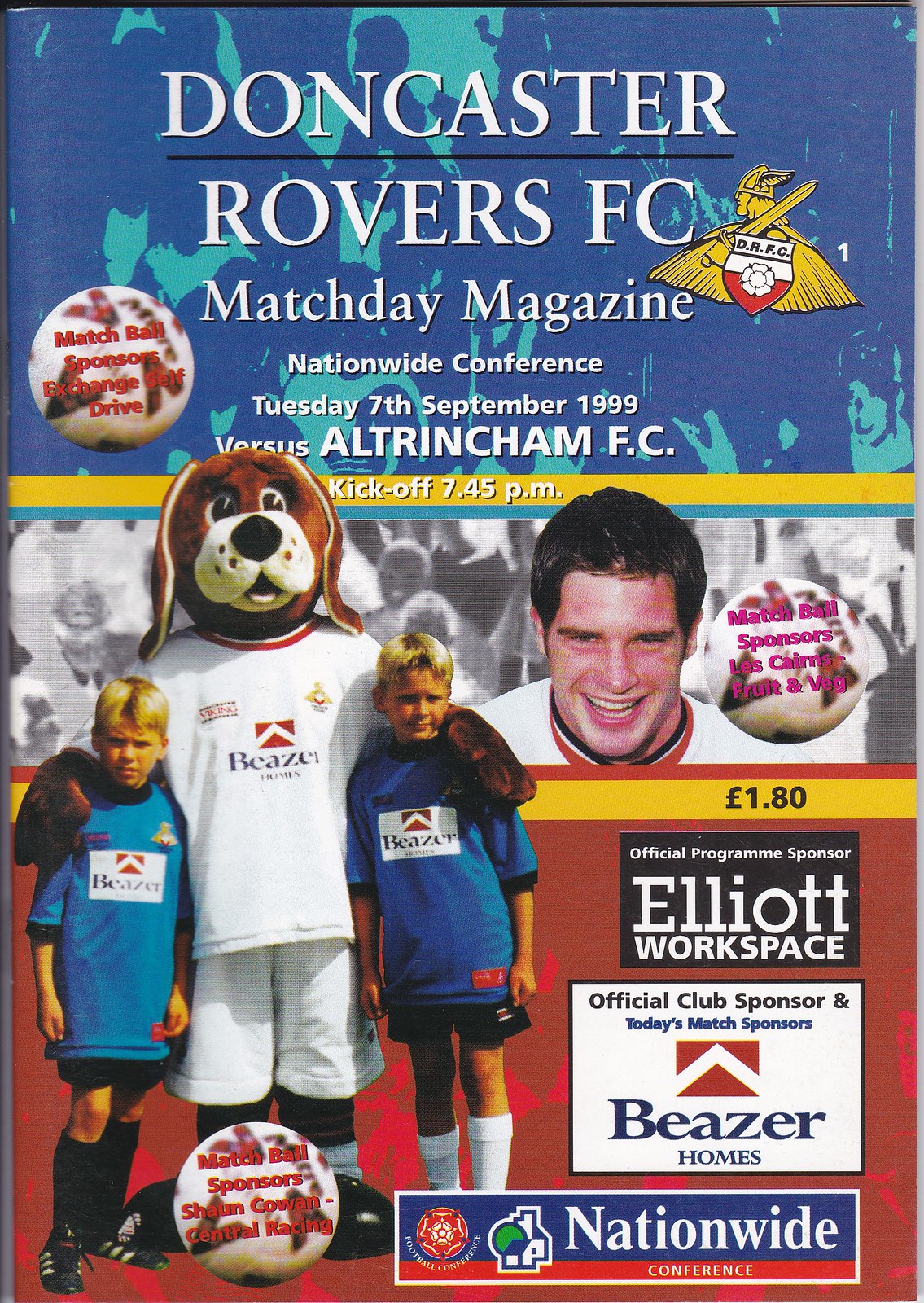The cover of the Doncaster Rovers FC match day magazine from Tuesday, September 7th, 1999, features a vibrant and engaging design typical of that era's promotional materials. Across the top, the title "Doncaster Rovers FC" is prominently displayed in a large, all-caps font, anchored by the club's logo, "DRFC," on the right side. Just below, it indicates the matchup against Altrincham FC, with a kickoff time of 7:45 p.m., set against a noticeable yellow background stripe.

Central to the cover is an eye-catching image of the team’s dog mascot, flanked by two young children, approximately 10 years old, all donning shirts emblazoned with "Beezer," the official sponsor. This trio stands out against the vivid backdrop and exudes team spirit. Additional sponsorships feature prominently in the bottom right corner, including "Official Club Sponsor" and "Today’s Match Sponsors" noted as Beezer Homes, emphasizing the community and commercial backing of the club.

The magazine also serves as a mini-poster, with the lower section showing various player images, enhancing its collectible appeal. Alongside the imagery are details of the "Nationwide Conference" and a mention of "Match Ball Sponsors Exchange Self Drive” on the left side, adding to the comprehensive information readily available for fans and readers. All these elements come together to create a detailed and nostalgic snapshot of a match day in 1999.